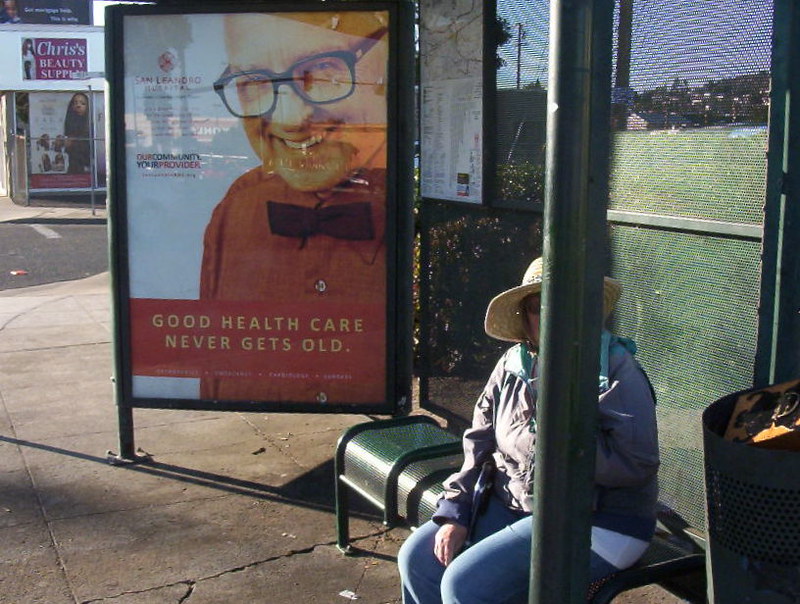This full-color photograph depicts a daytime street scene in an urban area, centered around a bus stop with a dark green, mesh-backed bench. A woman, wearing tight jeans, a light denim jacket, a straw hat, and sunglasses, is seated on the right side of the bench. However, a green pole obstructs much of her face and body. She appears to be waiting for a bus, suggesting a slightly cool day. Adjacent to her, on the bus stop structure, is a small billboard featuring a middle-aged man in black glasses, a bow tie, and a burgundy shirt. The advertisement reads, "GOOD HEALTH CARE NEVER GETS OLD" in bold yellow letters. The sidewalk beneath the bench is cracked, and sunlight illuminates parts of the ground. Nearby, there is a dustbin, and across the street, a small building housing Chris's Beauty Supply is visible. The urban character of the area is highlighted by these details.